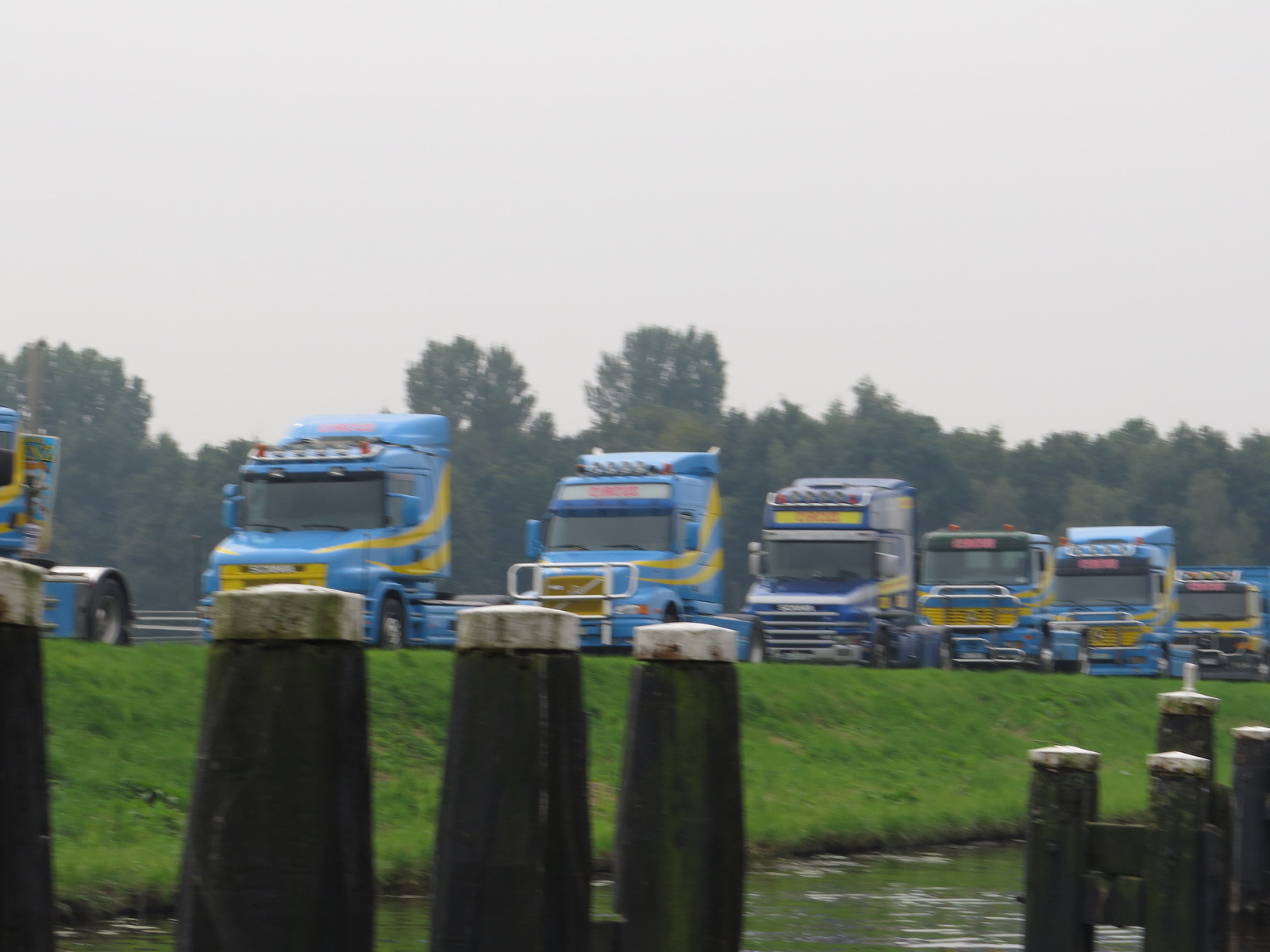In this blurry outdoor photograph taken from a pier or dock, eight thick, round, black bollards with white tops are seen emerging from a greenish lake or river; four of them stand alone on the left while the other four are connected by wooden beams on the right. Behind the water is a green grassy hill, which ascends to an unseen road where seven blue semi-truck cabs, each adorned with yellow stripes and a row of lights on top, drive closely together towards the viewer. Beyond the trucks, a dense row of trees can be seen, all under a gray, cloudy, and possibly rainy sky, contributing to the overall blurred and hazy atmosphere of the scene.